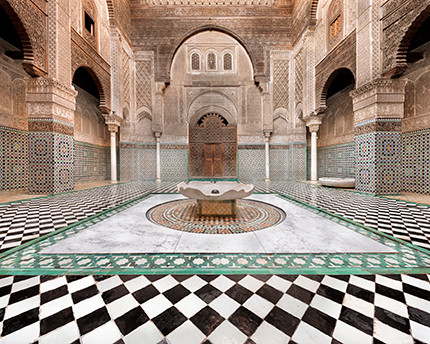The image captures a grand and ornate entrance hall, reminiscent of a Victorian-era structure with a touch of castle-like elegance. The walls are made of a mix of tan, brown, white, and goldish bricks, adorned with intricate mosaic tiles up to about eight feet high. At the forefront of this majestic space, there are three white pillars on each side, flanking a central golden door topped with three arched windows. The ceiling features a detailed tiling in darker shades of brown, gold, and gray.

The floor is primarily covered in an alternating black and white diamond-shaped tile pattern, contributing to the room's opulent atmosphere. The centerpiece of the floor is an elaborate, multicolored circular rug layered with a smaller, more vibrant turquoise and red-orange tiled section that surrounds a striking focal point—a large, ornate fountain resembling an open concrete flower. Latticework of green patterns surrounds this circular feature, adding to the complexity and beauty of the design.

The space is further framed by several grand archways that enhance the room's open and airy yet regal aesthetic. Overall, the hall exudes a sense of timeless beauty and detailed craftsmanship, with every element contributing to its breathtaking grandeur.